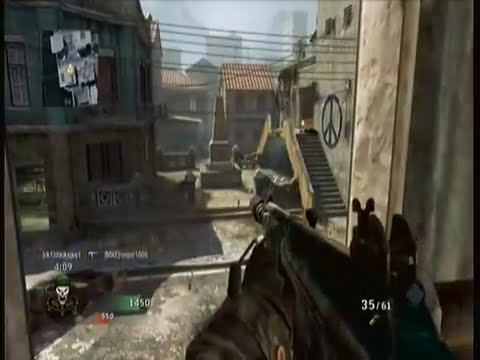The image appears to be a screenshot from a first-person shooter video game, likely from around 20 years ago, judging by the 4x3 format, suggesting it was played on a CRT monitor. The scene is set in a dilapidated, rundown neighborhood, possibly reminiscent of the Middle East based on the game's depiction style. The player is framing the shot through a window, with their character's hands holding a machine gun pointing out into the environment. The neighborhood features old, dilapidated apartment buildings, one of which has a tall, narrow staircase leading up to the front door, and a large black peace sign spray-painted on the wall next to it. Telephone wires hang loosely from the tops of the buildings. The ground and sidewalk are littered with rubbish and other debris. The heads-up display (HUD) includes a top-down map in the upper left-hand corner, a kill list on the right, and an ammo counter on the lower right. The overall scene conveys a sense of neglect and decay.